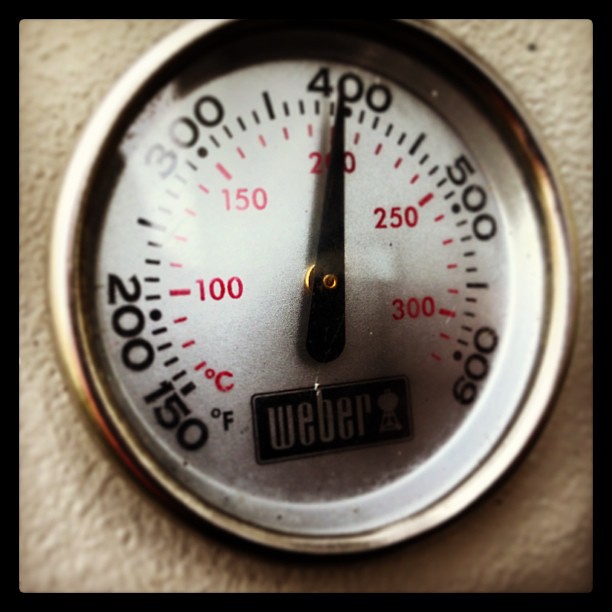This close-up image showcases a Weber grill thermometer, currently unattached and placed on a stucco-like surface. The thermometer, resembling a large metal button, features a prominent metal rim encircling a silver-white clock face. Black hash marks and numeric indicators of temperature in Fahrenheit adorn the outer edge, ranging from 150°F to 600°F on the far right. Inside, red hash marks and numbers denote Celsius temperatures, spanning from 0°C to over 300°C. A distinct black pointer indicates the temperature, and "Weber" is printed at the bottom against a black background. This precise and sturdy instrument embodies the quality associated with Weber products, essential for any barbecue enthusiast.